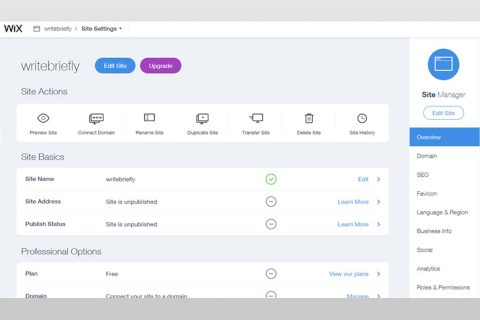The image depicts a comprehensive user interface of a Wix web page management dashboard with detailed elements:

The top section features a dark grey bezel. On the left-hand side of the bezel, the word "Wix" appears in black font. Just below, there's a rectangular button accompanied by grey text that reads "write briefly," and a grey arrow pointing to "site settings" written in black.

Beneath this, a light blue area with grey undertones bears the text "write briefly." Adjacent to this, there are two oval buttons: one dark blue with white text "edit site" and the other purple with white text "upgrade."

On the far left, the label "site options" is displayed in black. Below this is a large white rectangle with black-aligned text and several icons: an eyeball icon labeled "preview," a chat icon, a square labeled "connect domain," a folder with an eye and a truncated label "file name something." This section also features icons and labels for "duplicate site," a monitor with bands, "transfer site," a trash can labeled "delete site," and a clock icon labeled "see history."

On the right, within a blue circle, there's a white square with lines, labeled "site manager" in bold and regular black text. This includes another oval button with a blue border and text "edit site."

Back to the left, the "site basics" section is housed in a new white rectangle with bold black header text. Below, there are three items, each with a circle icon (two grey with a line and one green with a check mark) and hyperlinked blue text:

1. "Site name" with a "write briefly" description and an "edit" link on the right.
2. "Site address," noted as "site is unpublished" with a grey circle icon, and a "learn more" link with an arrow.
3. "Publish status," also indicated as "site is unpublished" with a grey circle icon.

Further down is the "professional opinions" section, showing a white rectangle labeled "plan," followed by "free," and a circle icon with a minus. Next to it, the blue hyperlinked text "view our plans" with an arrow.

Following this, there's the "domain" section indicating "free connect your site to a domain" with a dark grey circle icon. Below this section is an entry that starts with an "M" but is cut off.

Under the "site manager" label, the sidebar shows that the "overview" section is selected, highlighted with white text on a dark blue background. The remaining sections are listed in black text, including: Domain, SEO, Fusion, Language and Region, Business Info, Social, Analytics, Policies, and Permissions.